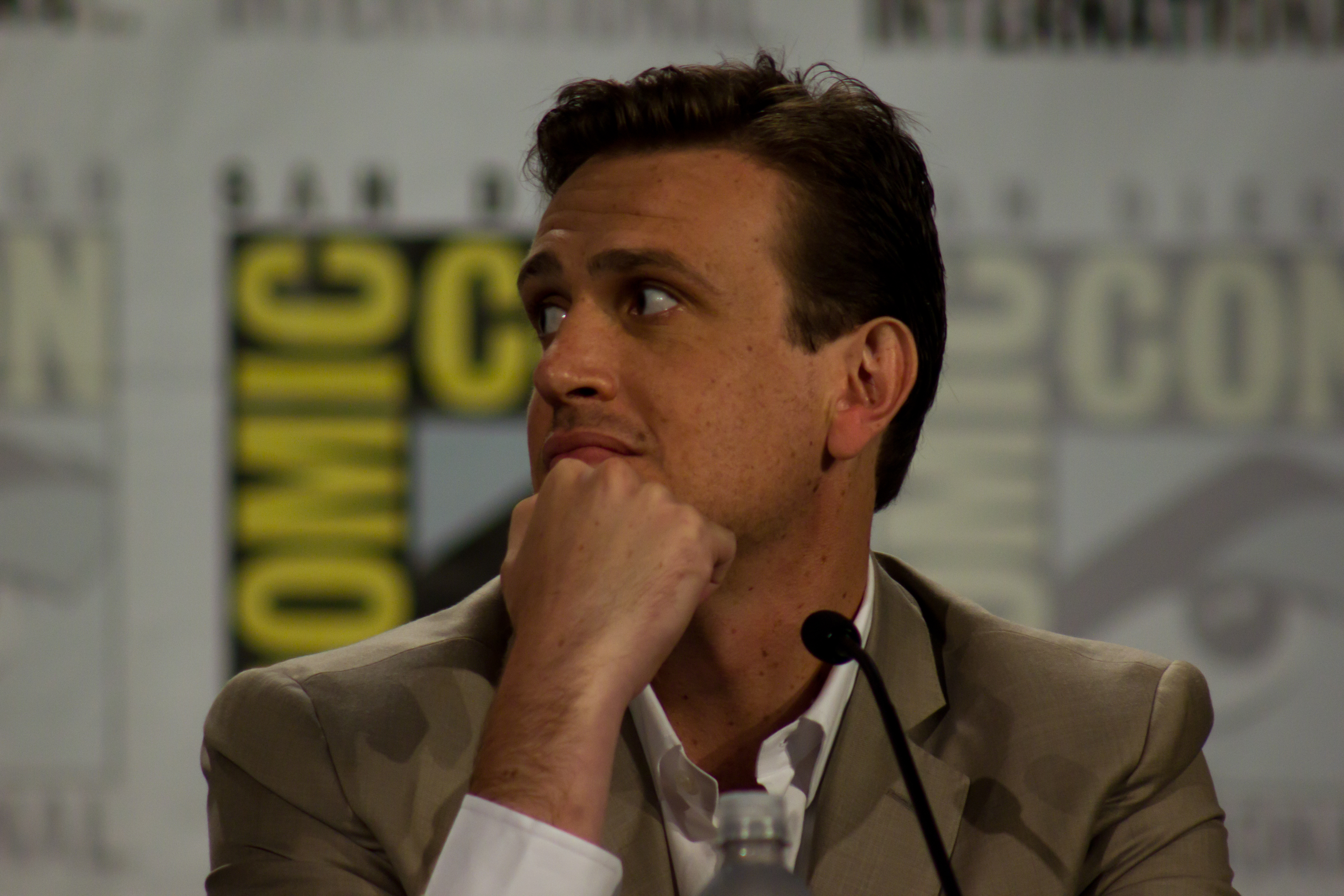The image features Jason Segel from the shoulders up, seated with a thin microphone in front of him. He appears thoughtful or concerned, with his right hand beneath his chin, supported by a closed fist, and his gaze directed towards his right shoulder. His short, dark hair is combed back, and he has a five o'clock shadow above his lip. He is dressed in a tan sports jacket over a white button-up shirt layered with a white t-shirt, with the top two buttons of the shirt unbuttoned, revealing the cuff of his sleeve. The backdrop is a repeating pattern with a Comic Con logo, featuring large yellow block letters on a slightly blurry white background, emphasizing the main focus on Segel. The well-lit and clear setting further highlights the details of his facial expression and attire.